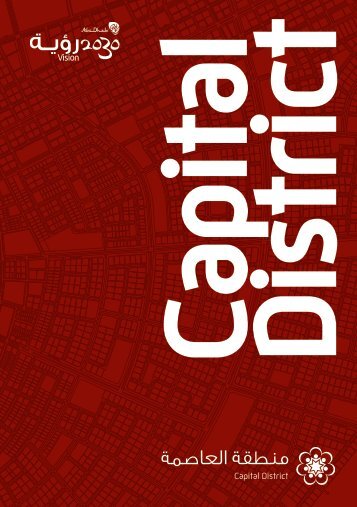The image depicts a dark red, map-like background, resembling an overhead view of a city with various subdivisions, roads, and blocks, possibly indicating housing or commercial spaces. Prominently displayed are several text elements:
- The top left corner features the large white text "Vision 2030".
- The right side of the image has vertical white text reading "Capital District".
- The bottom right corner repeats "Capital District" in white, accompanied by a small white flower-shaped logo with around 10 petals and a star-like center.

Throughout, there is additional non-English text, adding to the city's international feel. The layout suggests that this could be part of a city planning document or a visionary map for the future, potentially highlighting a "Capital District" reimagined for 2030.